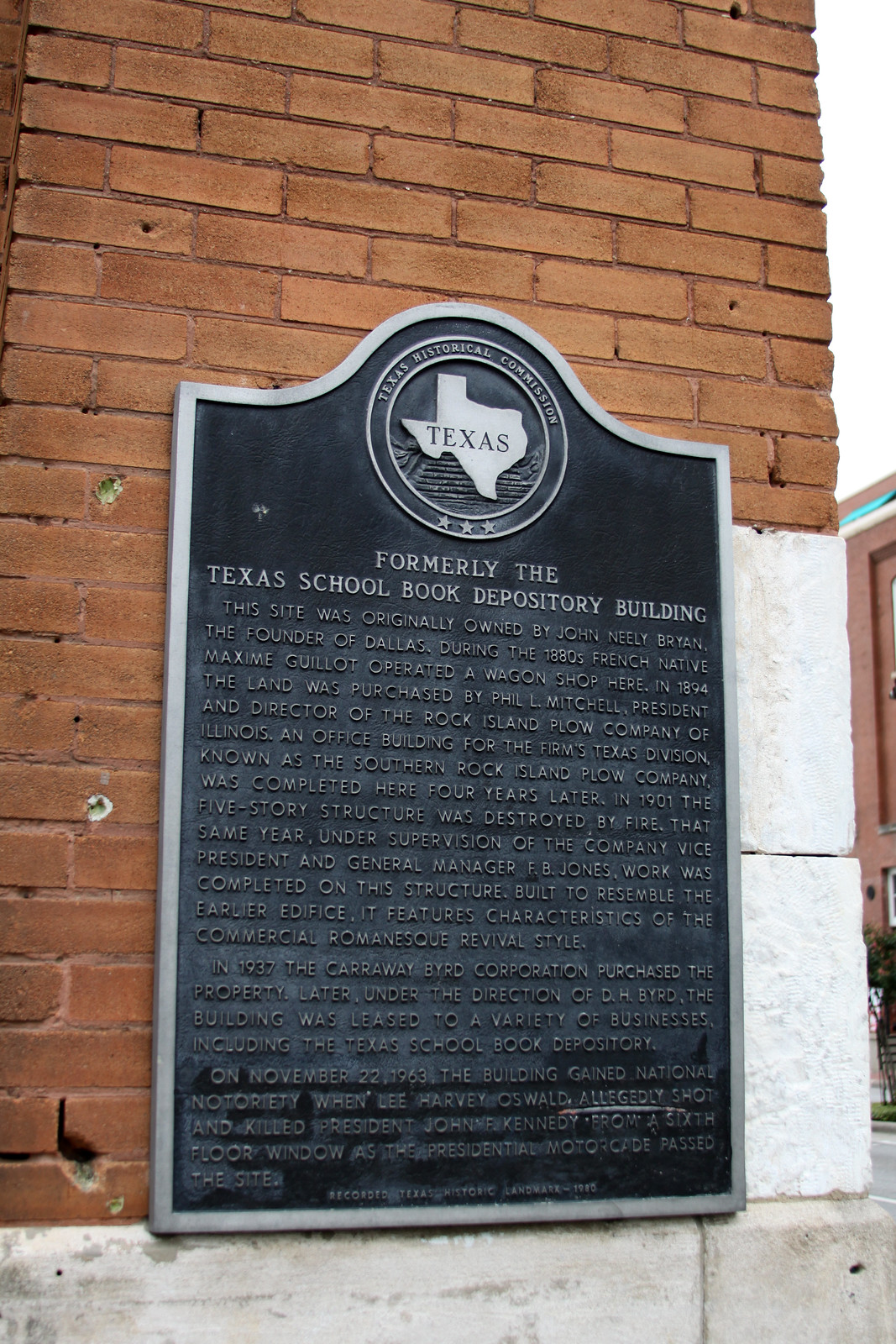This is a vertically aligned rectangular picture of a commemorative plaque attached to the brown brick side of a building, identified as the former Texas School Book Depository Building. The structure features a grayish-white stone base at the bottom, with two white stones prominently placed at the corner near the sign. At the top of the black, metal-faced plaque, bordered by gray, is a silver image of the state of Texas surrounded by a circular border with three stars along the bottom. Above the state image, "Texas Historical Commission" is inscribed, followed by three rectangular paragraphs of justified text beneath it. The raised gray print narrates the historical significance of the site, starting with its original ownership by John Neely Bryan, the founder of Dallas. It notes that during the 1880s, French native Maxime Gileot operated a wagon shop on the premises, and in 1894, Phil L. Mitchell purchased the land to build an office for the Southern Rock Island Plow Company. The building’s detailed history is encapsulated here, marking its importance in Dallas, Texas.